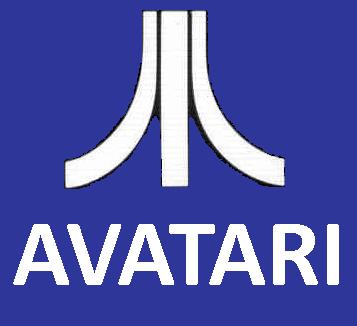The image depicts a dark blue, square logo that parodies the iconic Atari logo. Instead of "Atari," it reads "Avatari" in all capital letters, styled in white font. Above the text is a white symbol reminiscent of the classic Atari emblem. This symbol consists of a central vertical line flanked by two curving lines that resemble a slanted "J" and a slanted "L," which curl downwards, evoking a more artistic interpretation. The symbol and text are prominently displayed against the dark blue background, completing the minimalist and nostalgic design.